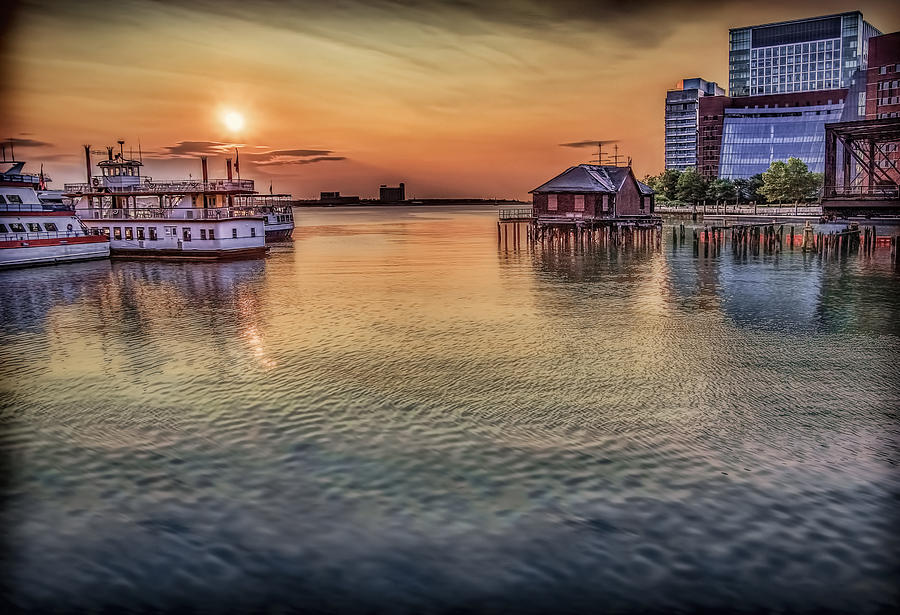This vivid photograph captures a serene waterfront bathed in the warm, glowing light of a setting sun, which has painted the sky in shades of orange and reflected its hues onto the water below. Ripples dance on the water's surface, interrupted here and there by patches of blue. On the left side of the image, a cluster of large, white boats, possibly tourist vessels, are docked. One boat stands out with its distinctive red trim. Further to the left, a boat resembling a floating restaurant reveals chairs inside, adding to the lively waterfront scene. On the right side of the image, a small cabin sits on a dock, its lights suggesting it's inhabited. Behind this cabin, a larger building with many windows looms, its modern design featuring blue glass. In the distance, across the water, the silhouettes of another city are faintly visible against the vibrant sunset, adding depth to the tranquil yet bustling scene.